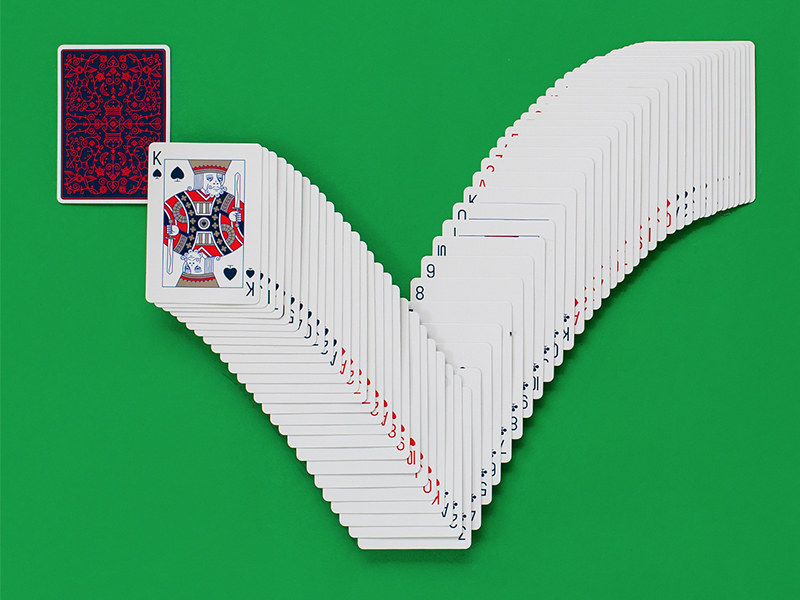This photograph showcases a meticulously arranged deck of playing cards artistically fanned out against a vibrant green background. The cards form a distinctive checkmark shape, with the left side of the checkmark positioned lower than the right. Highlighting the arrangement, one card in the upper left corner is turned face down, featuring a white border and a deep navy blue interior adorned with an intricate red floral design. This card also displays two ornate crowns, aligned vertically in opposite directions. At the pinnacle of the left side of the checkmark is the King of Spades, prominently visible. As the checkmark descends into a V-shape, several cards in the sequence—including an 8, 9, and 10—are clearly discernible. The arrangement then gracefully arches upward towards the upper right, completing the elegant and visually striking display.